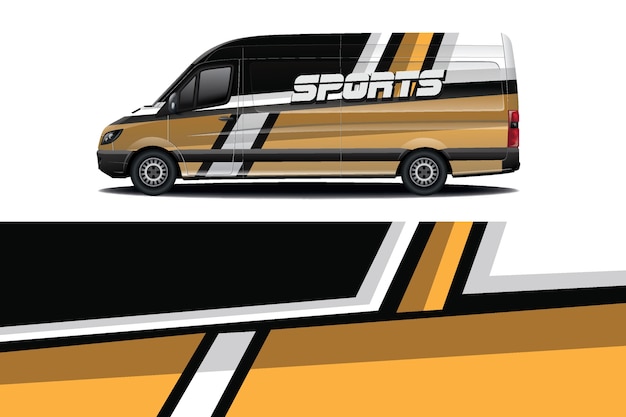The image features a delivery van positioned at the top half, facing the left and showcasing its left side profile. The van's sophisticated and ornate paint job is divided into sections with a gradient of colors and patterns. From the front to the middle, it displays a sequence of black, white, black, yellow, black and white stripes, and ends in white. The bottom half of the van predominantly features a brown color broken by a white line below the windows. The side of the van prominently displays the word "SPORTS" in bold white capital letters within a complex array of stripes that shift orientation from vertical to horizontal.

The van, characterized by a mix of black, white, brown, light brown, gray, and yellow hues, includes black tires and gray rims. Notable details such as the left headlight and red tail light are visible. Beneath the van within the image is a geometric pattern made up of four trapezium shapes with the upper left in black, upper right in white, and the lower two in yellow. Additionally, there's a rectangular section at the bottom part of the image, visually echoing the van's striped pattern but in a zoomed-in view for detailed inspection of the gradient and design elements.